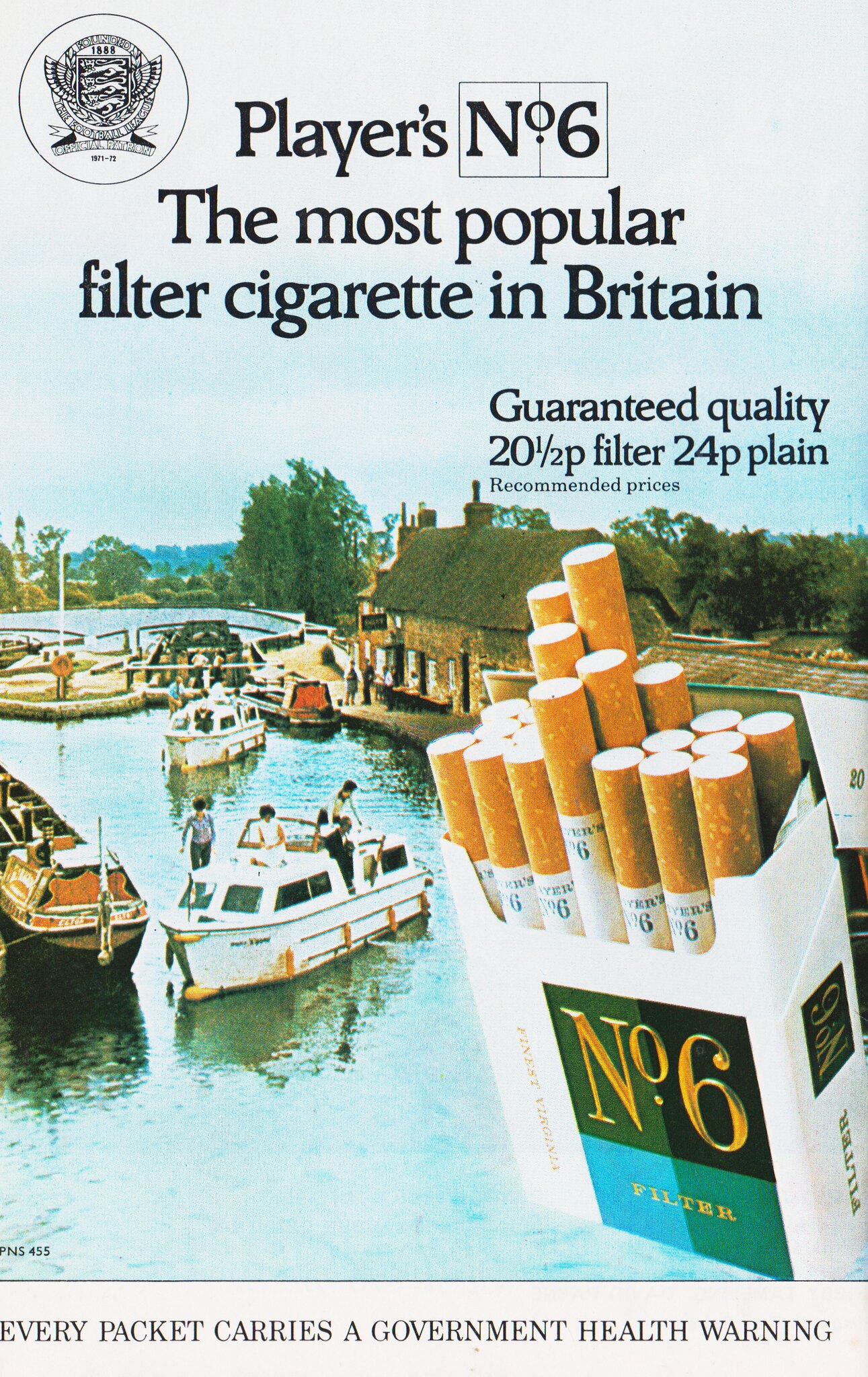This advertisement, likely from a magazine, prominently features an open pack of Player’s Number 6 filter cigarettes on the bottom right side. The pack, with about six cigarettes protruding slightly further than the rest, is set against a picturesque background of boats in a marina. The boats, some occupied by people, navigate through a narrow canal lined with trees, brown buildings, and docking stations. The sky above is overcast, enhancing the crisp blue of the water. In bold black letters at the top, the ad reads, "Player's Number 6 - The Most Popular Filter Cigarette in Britain." It also assures "Guaranteed Quality," and lists prices: "2.5 P filter, 24 P plain," with a note in small lettering, "recommended prices." At the very bottom, in all-capital black letters, it warns, "Every packet carries a government health warning."